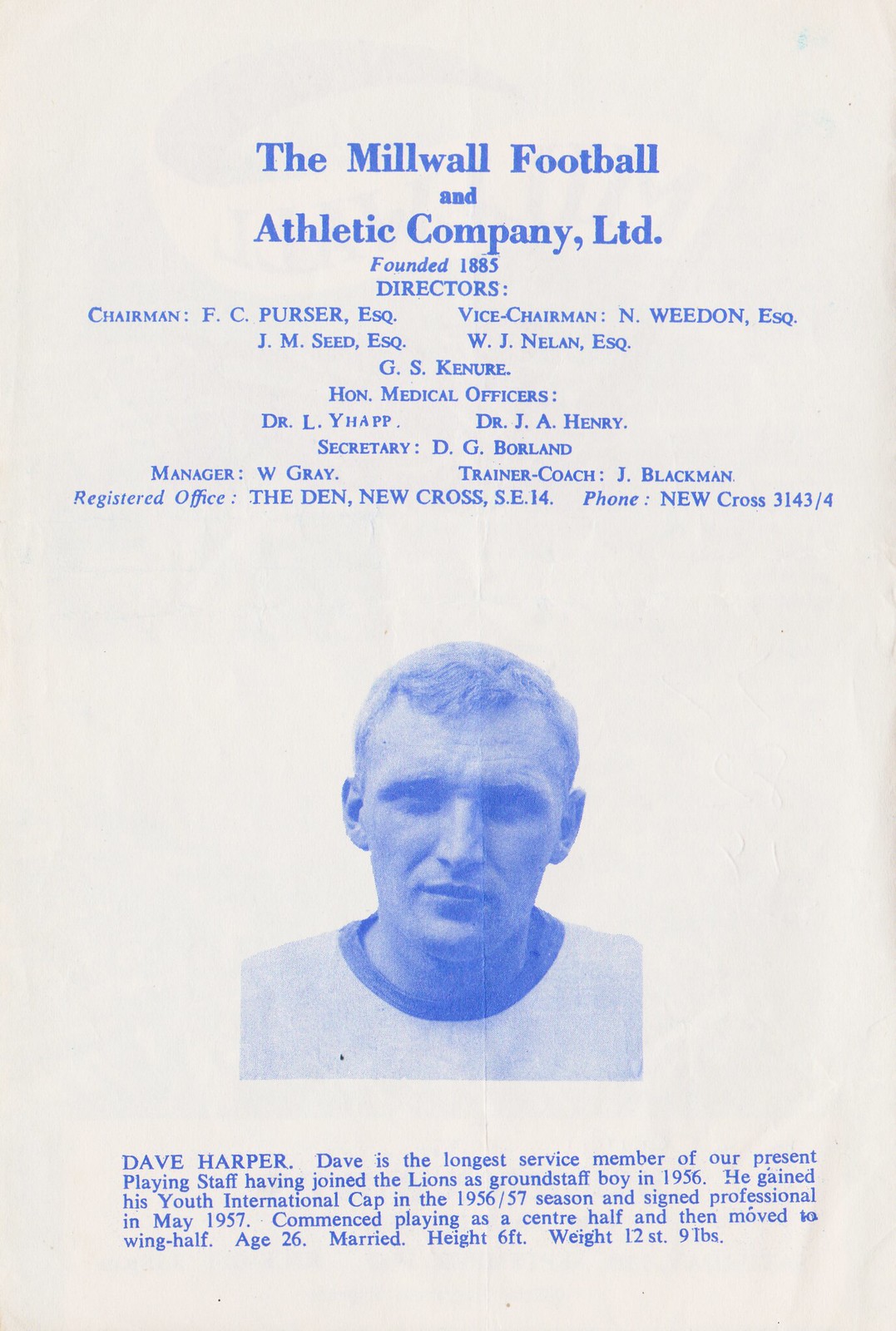This photograph captures an advertisement or flyer for the Millwell Football and Athletic Company Limited, founded in 1885. The flyer features bold blue letters on a white background with a faded blue photograph. At the top, the text reads "Millwell Football and Athletic Company Limited, founded 1885." It follows with a list of directors and officials: Chairman F.C. Purser Esquire, Vice Chairman N. Weedon Esquire, J.M. Seed Esquire, W.J. Nellon Esquire, and G.S. Kenyor. The Honorary Medical Officers listed are Dr. L. Yehoff and Dr. J.A. Henry, followed by Secretary D.G. Borland, Manager W. Gray, and Trainer Coach J. Blackman. The registered office details are "The Den, New Cross, S.E. 14" with the phone number "New Cross 3143-4".

In the center of the page is a blue-tinted photograph of a man identified as Dave Harper, a Caucasian male in a white shirt with a colored neckline, characterized by his short hair and squinting eyes. The text under the photograph notes that Dave Harper is the longest-serving member of the present playing staff, having joined the Lions as a ground staff boy in 1956. He gained his youth international cap in the 1956-57 season and signed professionally in May 1957. Initially playing as a center half, he then moved to wing half. Further details include his age (26), marital status (married), height (6 feet), and weight (12 stones, 9 pounds).